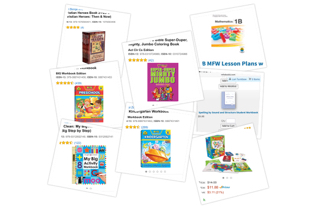The image depicts a collection of children's educational products, with a focus on books and possibly board games. The products are organized into eight distinct squares, each slightly overlapping and arranged at various diagonal angles, forming a visually engaging pattern. Three squares are positioned on the left, two in the upper center, and three more on the right. Each square contains vertically aligned information, despite the cards themselves being angled. The details include the product name, the number of reviews, and a small icon representing the item. One notable product in the upper right corner is labeled "MFW Lesson Plans." The overall design suggests a layout aimed at first or second-grade educational materials, presented on a clean, white background that seamlessly blends into the surrounding space. The image aims to convey a sense of order and information about various educational tools available for young learners.